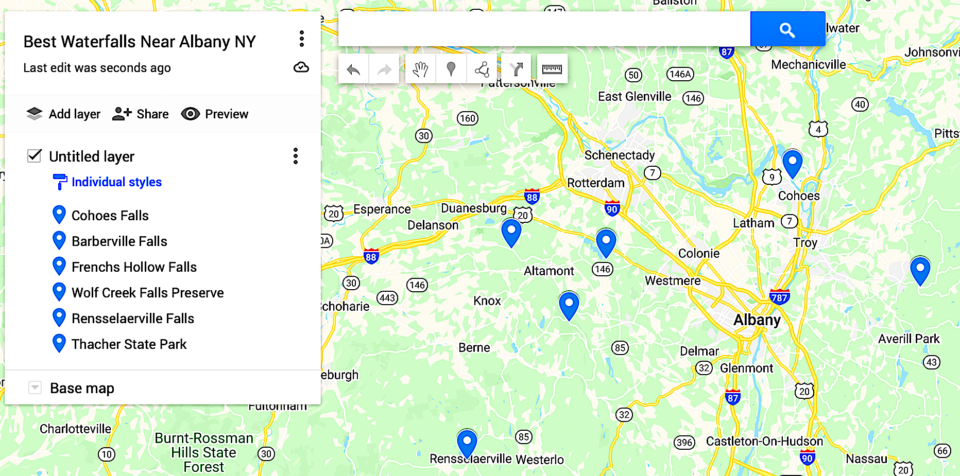Detailed Caption: 

The image portrays a highly detailed map focused on the best waterfalls near Albany, New York. Dominating the left side of the image is a tall, vertical white rectangle labeled "Best Waterfalls near Albany, New York" in black font. This section also includes options like "Last edited seconds ago," "Add Layer," "Share," "Preview," and "Untitled Layer." 

The map itself features a network of green and light brown-yellow colors representing the natural landscape and streets or highways. Distributed across the map are numerous blue pins indicating the locations of notable waterfalls, such as Echo Falls, Barberville Falls, French's Hollow Falls, Wolf Creek Falls Preserve, and Rensselaerville Falls, among others.

In addition, locations like Thatcher State Park and several other waterfalls are marked. The term "Individual Styles," also in blue, suggests customizable views for each pin. At the top, a search bar is present with a blue button featuring a magnifying glass icon. The toolbar includes a back button, a forward button, a hand button, a pin button, an unknown button resembling a circle-line pattern, and another button likely for changing directions. The exact function of a final button, noted as the "pet button," remains unclear. The overall interface is characterized by white backgrounds and black text, maintaining a clean and organized look.